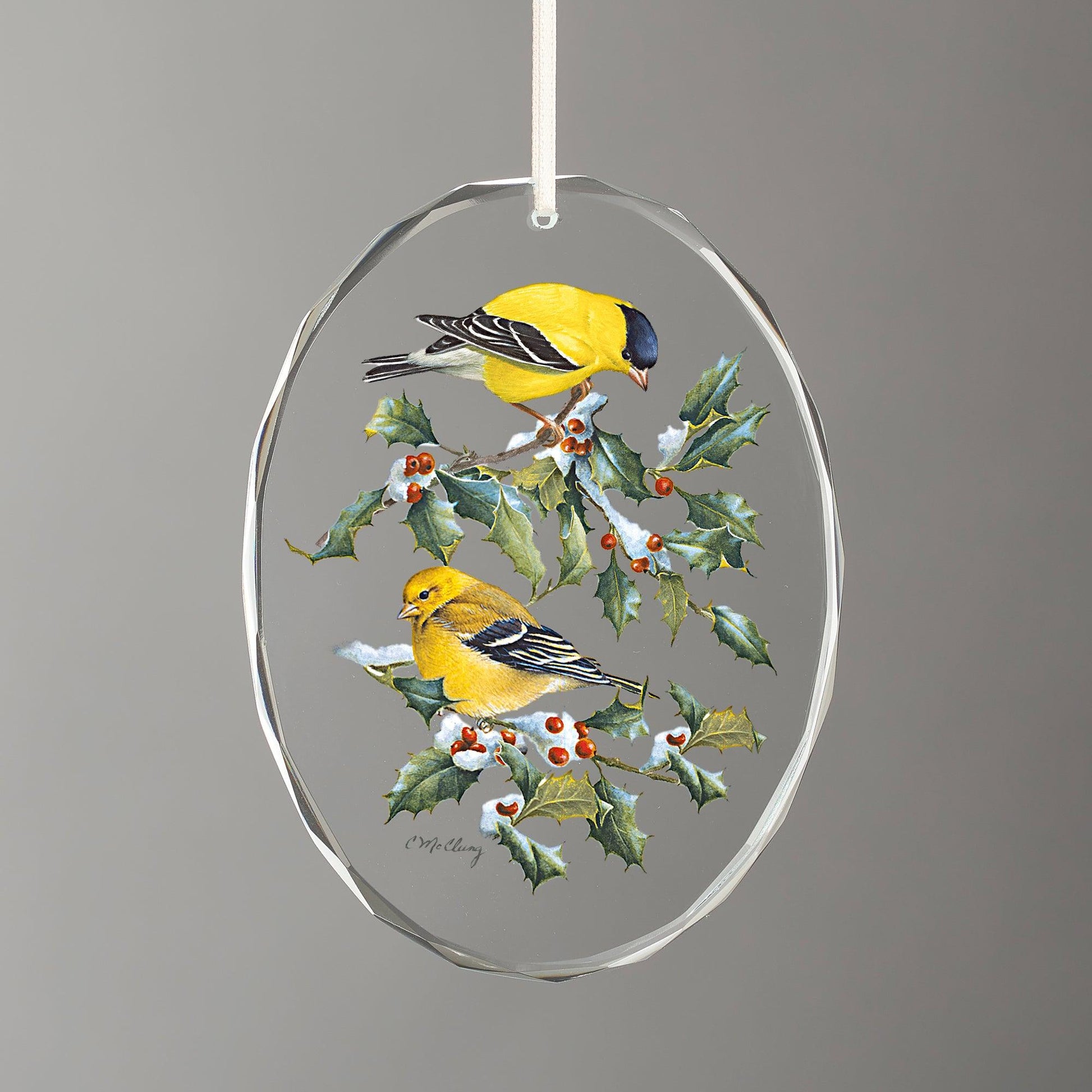In this vertical rectangular image, set against a dark gray background, we see a clear plastic or glass decoration hanging centrally from a white ribbon. The overall shape of the decoration is an oval. Surrounding it is a silver-gray metal hoop with slightly bent, curvy edges that gives the piece an intricate, artistic feel. 

Inside this oval, there are intricately painted depictions of birds and foliage. At the top, a yellow bird with a black head, black wings, and black tail feathers perches on a branch adorned with green holly leaves and red berries, dusted with a touch of snow. This bird is looking downward. Below it, another yellow bird with black wings but no black head is positioned on a similar branch also decorated with leaves, red berries, and a hint of snow. The meticulous details and vibrant colors make this hanging decoration resemble a delicate Christmas ornament.